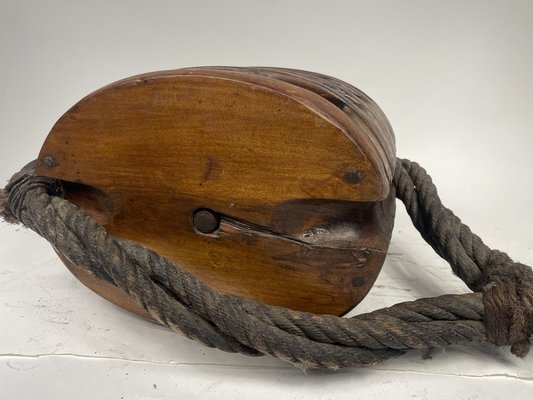This photo features a dark brown, ovular wooden object, possibly a nautical component. It's positioned horizontally against a solid white background with a subtle surface crack. Two thick, dark ropes extend from either side of the wood, with the left section frayed and looping across the front to knot with the right section. The ropes appear worn and are darker in color. The wood itself has visible knots and a screw in the center, adding to its intricate details. The composition highlights the contrast between the dark, textured materials and the pristine white background, making the wooden object and ropes stand out vividly.